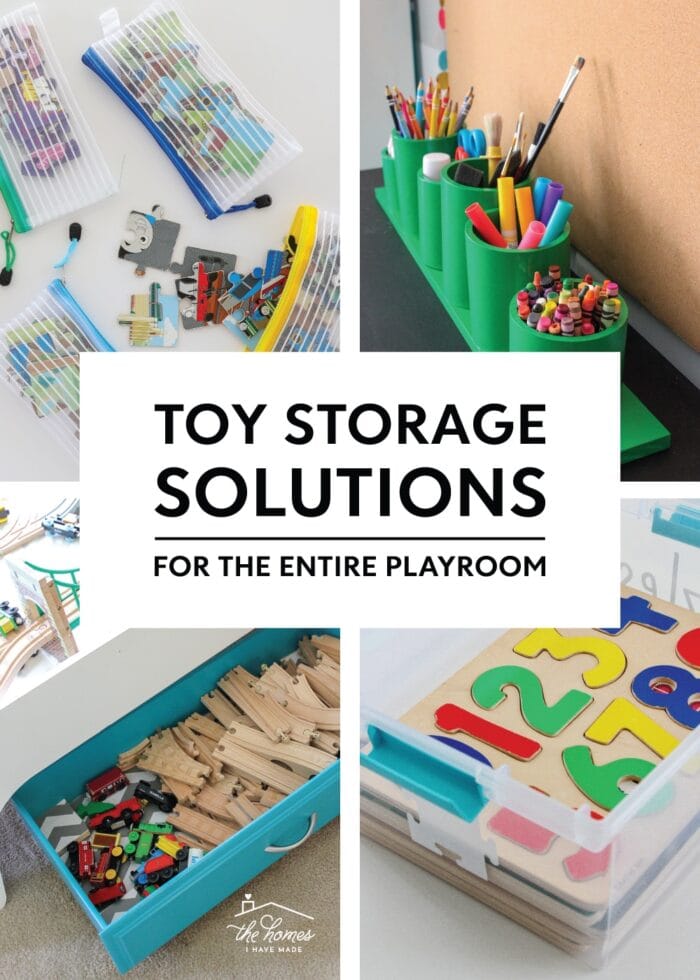The advertisement features a vertically aligned rectangular image divided into four sections, depicting a vibrant and organized children's playroom. In the center, a white horizontal rectangle with black text reads, "Toy Storage Solutions" and "For the Entire Playroom," underlined for emphasis. 

The top-left section displays several color-coded, zippered bags containing various art supplies like pencils and crayons, with some items spilling out, suggesting easy access and child-friendly organization. The top-right section showcases a green multi-cup stand filled with assorted writing and craft materials, including markers, paintbrushes, colored pencils, scissors, and glue sticks, all neatly arranged in green containers.

In the lower-left corner, a partially pulled-out blue drawer reveals wooden train track pieces and toy cars, emphasizing tidy and playful storage. The lower-right section features a clear storage bin with blue handles, containing colorful wooden puzzles with numbers 0 through 9, set against a natural wooden backdrop.

Additionally, on the lower left-hand picture, there is a logo of a roof with a chimney, accompanied by the scripted text "The Homes," suggesting the brand behind the storage solutions. This detailed, eye-catching poster effectively highlights practical and appealing organizational options for a well-kept playroom.